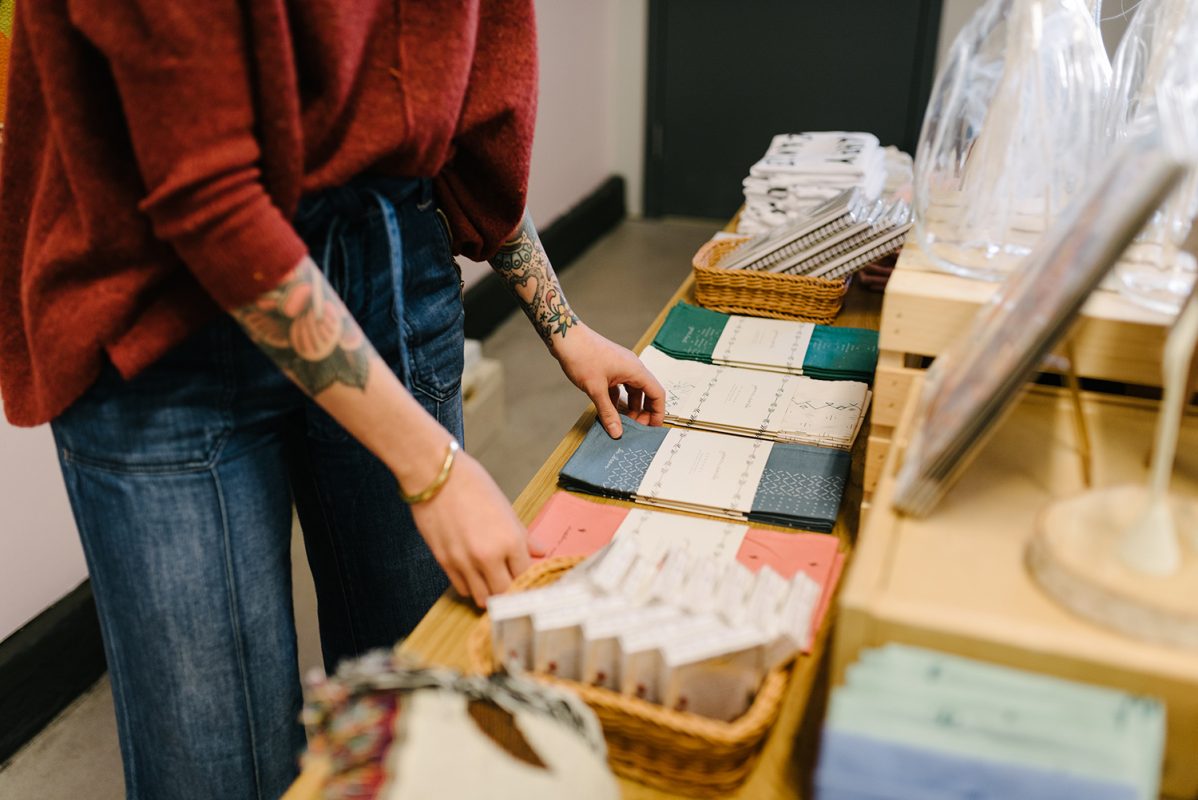This photo captures a person wearing a maroon, long-sleeved sweater with the sleeves pulled up, revealing tattoos on both arms; the tattoo on the right arm is of flowers. The person is also wearing dark denim jeans and a gold bracelet. They stand in front of a table that appears to be set up for a business or a class, organizing various products. The table holds notepads in different colors—green, pink, blue, and white—as well as pieces of fabric, some tablets, and baskets filled with what look like cards or additional notepads. In the background, there’s a light brown case with what might be a magazine or a photo on display, though it is out of focus. There is also an open door leading out of the room, and out-of-focus items are scattered around. The woman's face is not visible, but her focused action suggests she is preparing for an event or presentation.